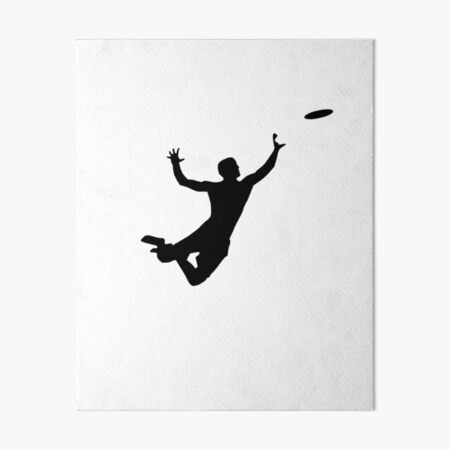The image features a dynamic silhouette of a man against a stark white background, capturing a moment of intense action. The man's shadow is entirely black, lending a dramatic contrast to the scene. He appears to be high up in the air, either leaping or flying, with his knees bent backward and both arms raised skyward. His left hand is open, fingers splayed in a C-shape, poised to catch a frisbee also depicted as a black silhouette. The overall composition, with the black-and-white color scheme, the blurred quality, and the resemblance to a picture of a piece of paper, conveys a sense of motion and excitement, making it suitable for use in art or advertisements.